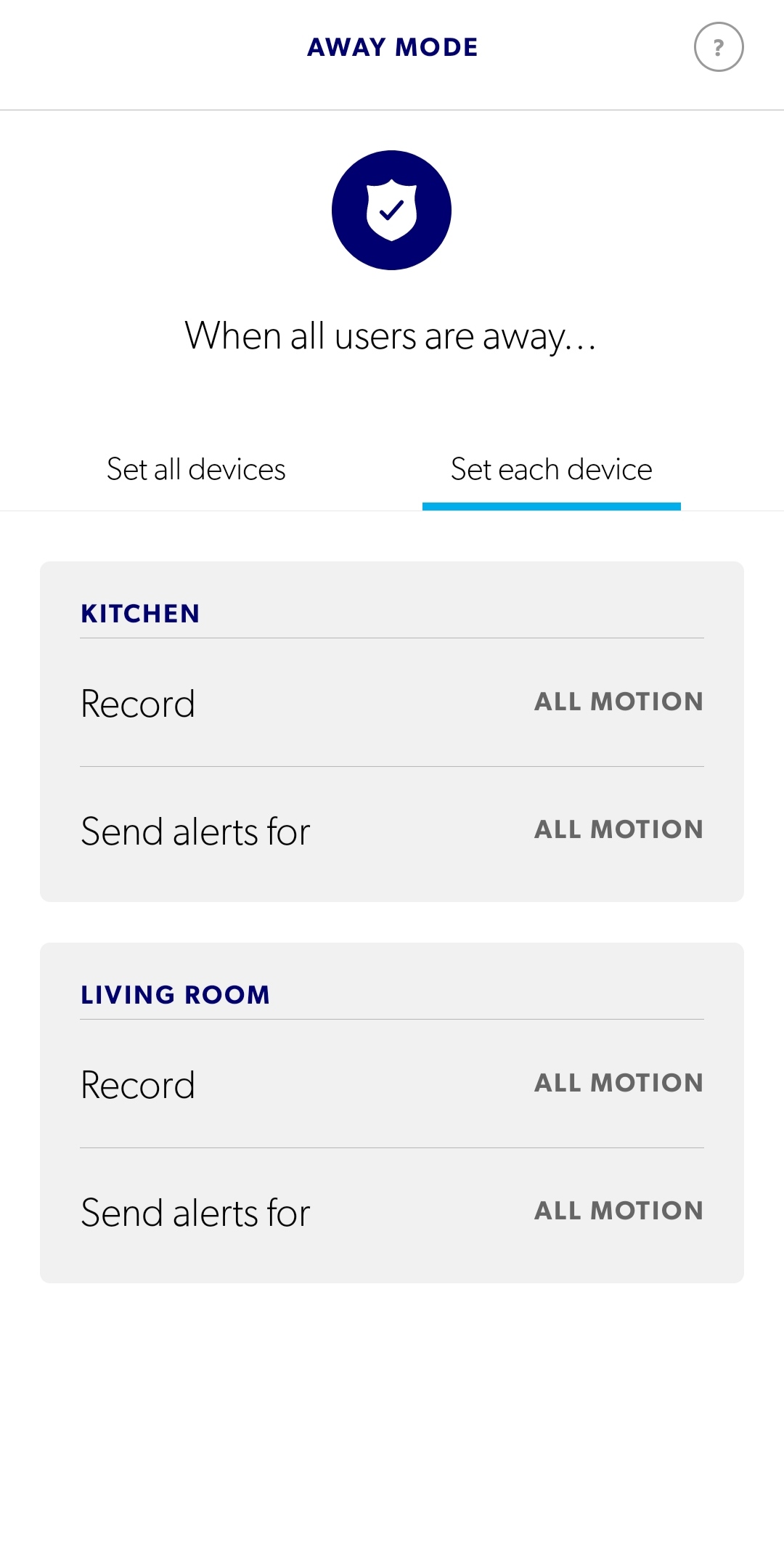The image is a screenshot from a security app on a cell phone, prominently displaying an "AWAY MODE" screen in blue, capital letters. To the right of the "AWAY MODE" text is a small white circle containing a question mark, indicating help or additional information. Below this title is a thin, horizontal gray line stretching across the screen.

Further down, there is a navy blue circle with a white shield and a checkmark in its center, signifying protection or successful activation. Below this icon, the text reads, "When all users are away..." Two selection options, "Set All Devices" and "Set Each Device," are presented next. "Set Each Device" is underlined in blue, indicating it is the option currently selected.

The interface then shows settings for two rooms, each contained within a light gray rectangular box labeled "Kitchen" and "LIVING ROOM" in capital blue letters. For both rooms, there are options labeled "Record" with a selectable "All Motion" setting, and "Send Alerts For" with a "All Motion" option again. These settings allow users to configure the security actions for each room when the away mode is activated.